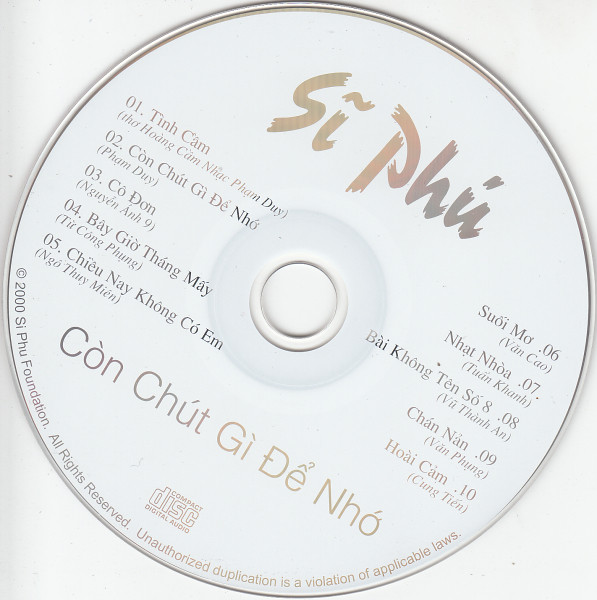The image depicts a music CD titled "S.I.P.H.U," easily identified by its predominantly white surface with a silver edge. The text on the CD is written in Vietnamese, clearly detailing the ten tracks included. On the left side of the disc are the first five tracks: "Teen Camp," "C-O-N-C-H-U-T-G-I-D-E-N-H-O," "C-O-D-O-N," "B-A-I-O-T-H-A-A-N-G-M-A-Y," and "C-H-I-E-U-N-A-Y-K-H-O-N-G." The right side lists tracks six to ten: "C-O," "E-M," "N-A-T-N-O-A," "B-A-I-K-O-N-G-T-E-N-S-O," and "C-H-A-N-N-A-N." The disc also features smaller text at the bottom reading "At Two Thousand Supreme Foundation All Rights Reserved." Despite its clean background and somewhat transparent, reflective lettering, typical for Compact Disc Digital Audio, the content is clearly structured and articulated, revealing the meticulous details of each track in Vietnamese, with hints of a reflective shine if held against the light.